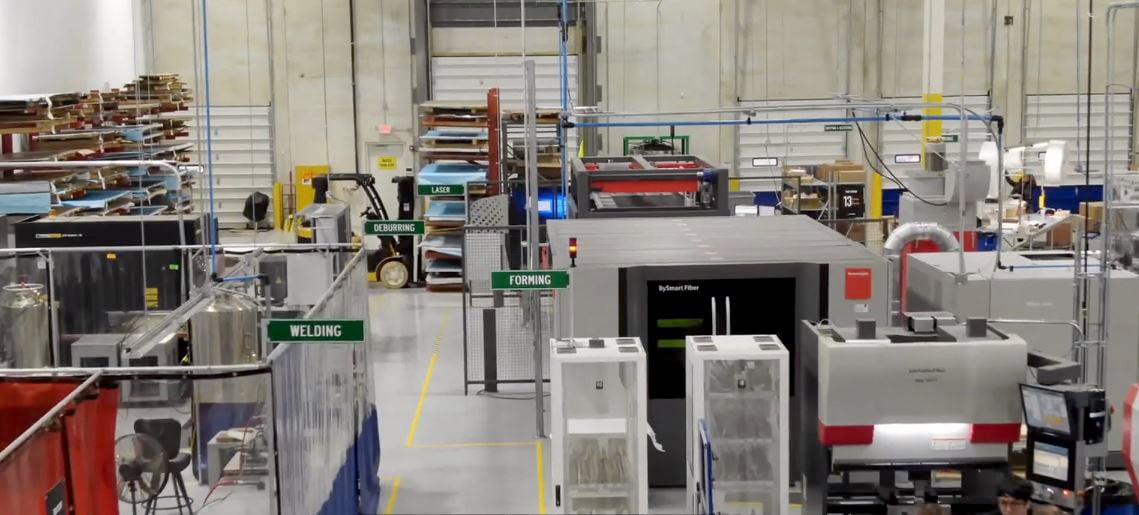This detailed photograph taken indoors at a sheet metal fabrication factory captures a bustling workshop environment filled with various machinery and equipment. Dominating the scene are labeled areas demarcated by green signs with white lettering, indicating distinct sections such as "forming," "welding," "deburring," and "laser." At the center, the "forming" area features a large piece of equipment resembling an airport X-ray machine, used for processing materials. Adjacent to the "forming" section, the "welding" area is enclosed by plastic curtains, designed to contain debris. Down toward the left, a forklift is positioned under the "laser" sign, lifting a metal shelf likely loaded with metal sheets. The background includes white walls with corrugated garage doors and visible wooden pallets on the upper left. The image, taken from an elevated angle looking down, showcases rolling racks covered in plastic to protect their contents and cubicle-like workstations, one featuring a blue chair and fan. The overall ambiance is industrial, dominated by shades of gray, accentuating the factory setting where metal fabrication processes are in full swing.